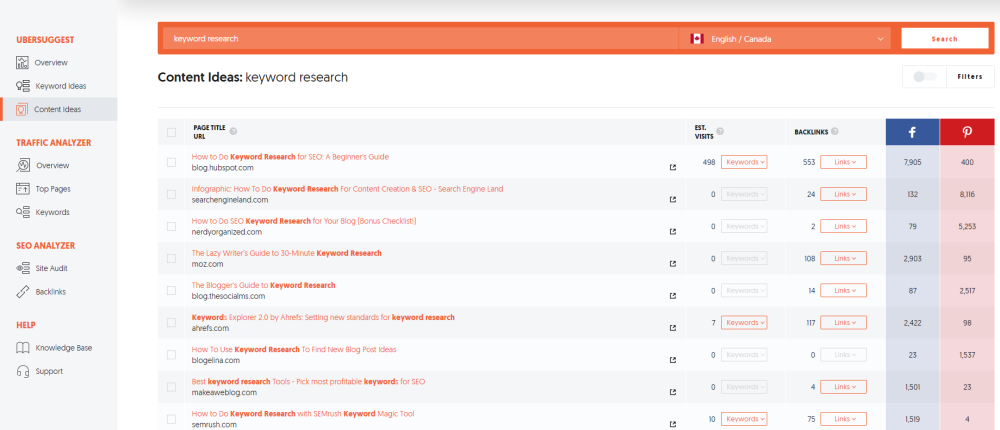The web page features a structured layout with a left column that categorizes various sections using distinctive orange headings and black subheadings. The topmost section is labeled "UserSuggest" (in a single word), followed by subcategories like "Overview," "Keyboard," and "Content Ideas," with "Content Ideas" actively selected, indicating the current page view. Further down, the orange heading "Traffic Analyzer" introduces subcategories such as "Overview," "Top Pages," and "Keywords." Below, "SEO Analyzer" marks another section with "Site Audit" appearing within brackets subsequently. The final section, titled "Help" in orange, includes "Knowledge Base" and "Support," each accompanied by relevant icons.

To the right, a prominent orange banner contrasts with the surrounding elements. Adjacent to this banner, a list titled "Keyword Research" sits beside a Canadian flag icon, which includes a dropdown menu suggesting an English (Canada) language option. A white search box is situated below, paired with headings in black for "Content Ideas" and "Keyword Search." Following these headings are nine vertical entries, though the specific content is unreadable. Flanking the entire right side of the page are traditional blue and red icons for Facebook and Pinterest, respectively, adding social media integration.